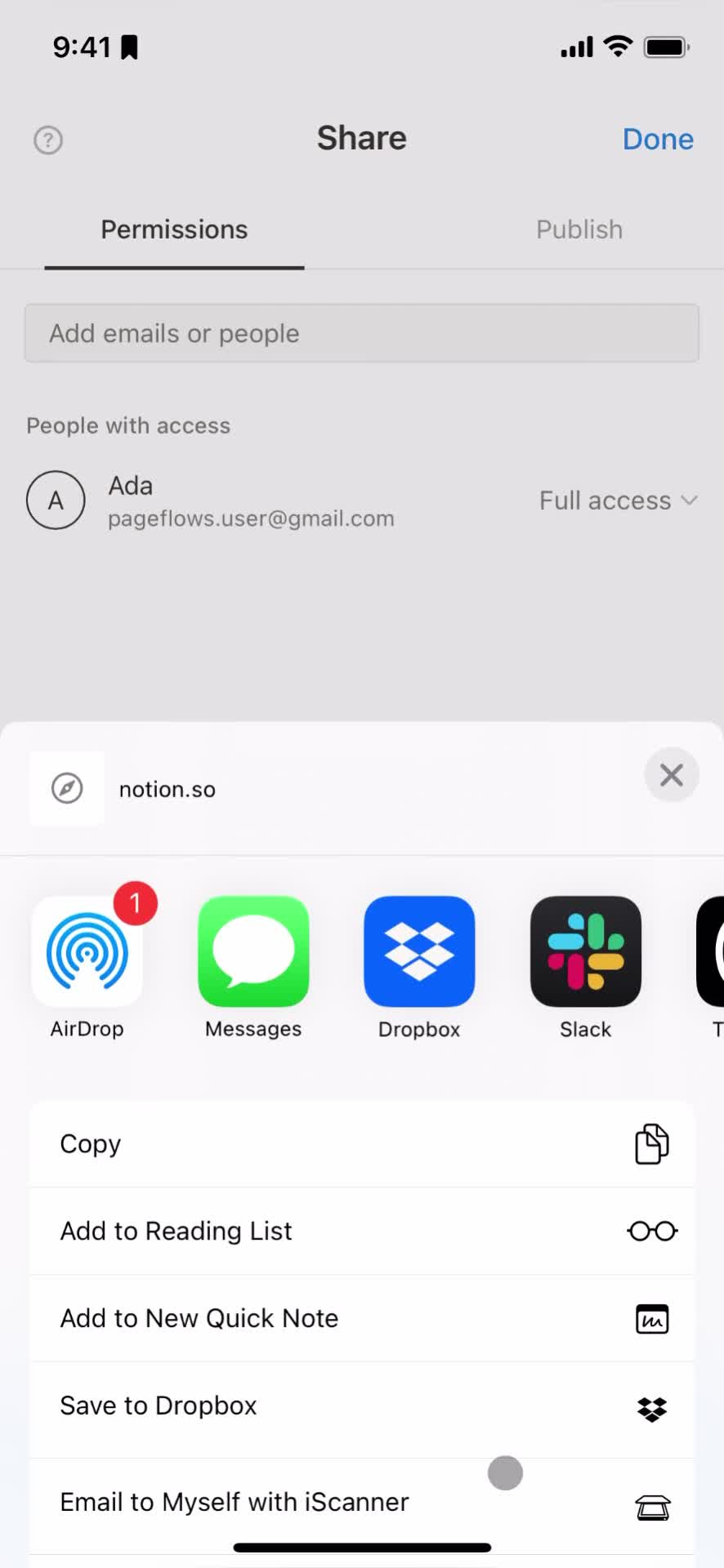The image is a screenshot from an iPhone, showcasing a particular screen with detailed interface elements. At the very top right of the image, the battery icon indicates a full charge. To the left of it, both the Wi-Fi signal and the phone signal strength icons are also at full bars. On the top left corner, the current time displayed is 9:41, accompanied by a bookmark icon.

Centrally at the top, the word "Share" is visible. Directly beneath it are two categories: "Permissions" on the left and "Publish" on the right. The "Permissions" tab is currently selected, highlighted by a darker color and a black underline, while the "Publish" tab appears grayed out.

Within the main section of the screen, there is a rectangular text box displaying the option to "Add emails or people". Below this box, a heading reads "People with access," listing a user named Ada with the email ageflows.user@gmail.com.

The bottom half of the image reveals a pop-up box. At the top left of this box, the text "notion.so" is visible. The pop-up contains several app icons in square shapes, including AirDrop, Messages, Dropbox, and Slack. Additional options displayed below these icons include "Copy," "Add to Reading List," "Add to Note," "New Quick Note," "Save to Dropbox," and "Email to myself with iScanner."